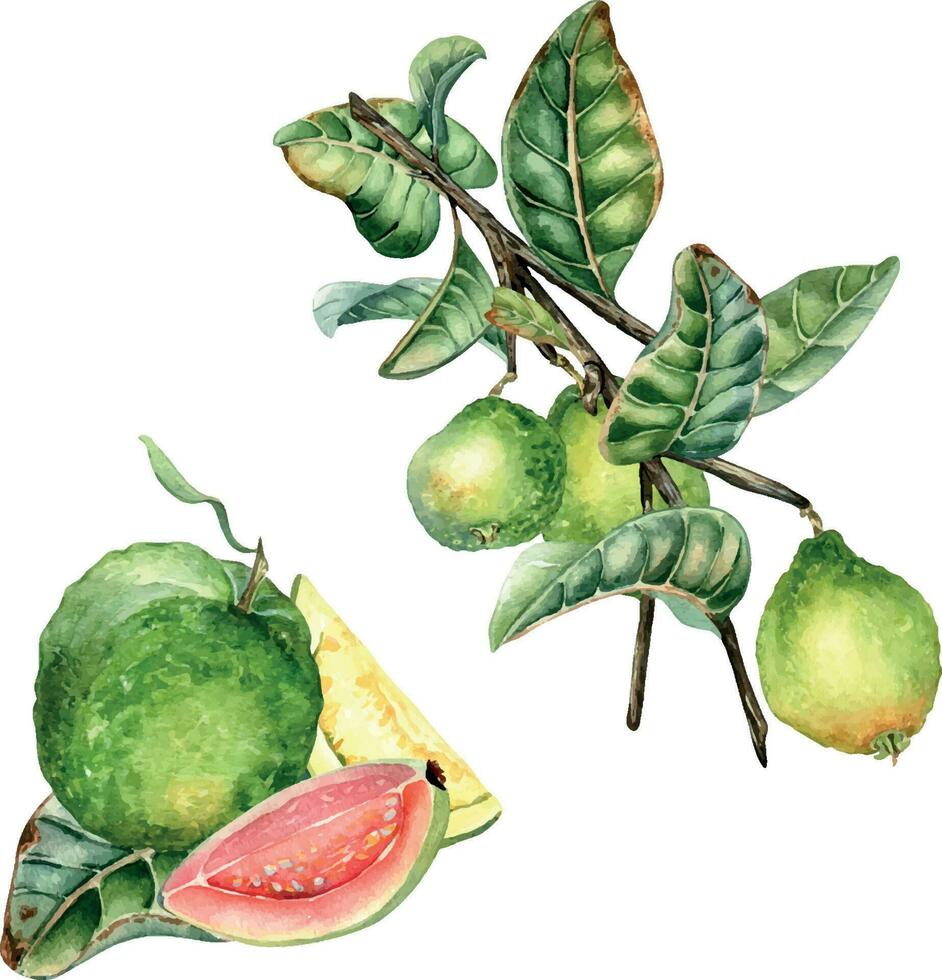The image displays a detailed artwork set against a pure white background, emphasizing the vivid colors of the depicted plants. Dominating the bottom left quadrant is a green fruit, likely a guava, with slices removed to reveal distinct sections—one yellowish, indicative of an unripe state, and the other pinkish, representing ripe flesh. Both slices contain small seed-like details. The upper two-thirds of the image features a branch with large green leaves and round, green fruits—presumably the same guava fruit in an uncut form. This mixed media piece, possibly created with watercolors and colored pencils, showcases the stages of the fruit's ripeness while the rest of the image remains unadorned, without any artist's signature.